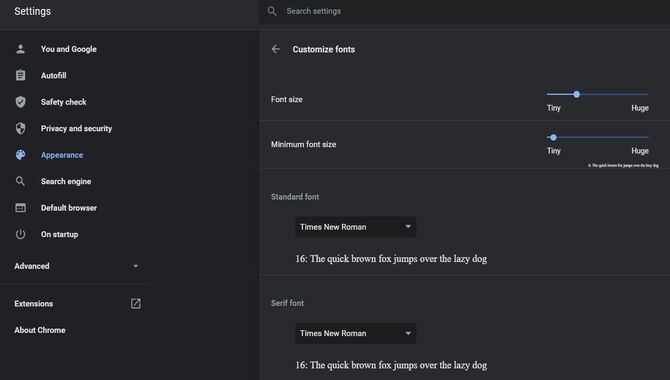Settings page of a web browser displayed. At the top, there's a grey bar labeled "Search Settings". On the left side, a column lists various options: "You and Google", "Autofill", "Safety Check", "Privacy and Security", "Bluetooth", "Appearance", "Search Engine", "Default Browser", "Start Up", "Advanced", "Extensions", and "About Chrome".

The interface is designed with clustered fonts, predominately grey, and the font size appears quite small. A bar adjusts the minimum font size, currently set to "Tiny". 

The standard font for the displayed text is "Times New Roman" at size 16, as shown in a grey rectangle with a sample text "The quick brown fox jumps over the lazy dog". 

The background of the settings page is a very muted grey, providing a subdued and simple aesthetic that emphasizes the text options and settings provided.